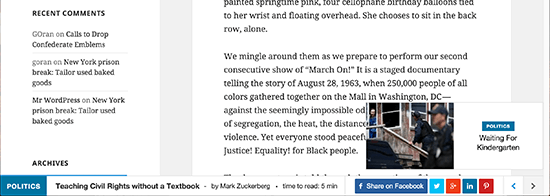This rectangular snapshot appears to be taken from an online article. The long side of the image runs horizontally from left to right. On the right-hand side of the image, there's a section labeled "Recent Comments," featuring several snippets:

1. "Go ran on calls to drop Confederate emblems."
2. "Go ran New York prison break."
3. "Taylor used baked goods."
4. "Mr. Woodpress on New York prison break, Taylor used baked goods."

These comments seem to pertain to the content of the article, though the full text is not visible. A partially readable paragraph begins with, "We mingle around them as we prepare to perform our second consecutive show of March on. It is a staged documentary telling the story of August 20th, 1963, when 250,000 people of all colors gathered on the Mall in Washington, D.C. against the seemingly impossible." However, this text is obscured by an overlay box that reads, "Waiting for Kindergarten," making the rest of the paragraph illegible.

At the bottom of the image, a banner runs across the width, providing additional information. It reads, "Politics: Teaching Civil Rights Without a Textbook" by Mark Zuckerberg. The image also contains various other boxes with different symbols, further hinting at the article's multi-faceted content.

This detailed caption encompasses the visible elements and partially hidden content of the image, providing a thorough description.